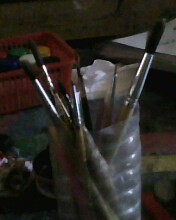The photograph captures a dimly lit indoor scene dominated by a deeply shadowed background. Slightly off-center to the right, a repurposed, ribbed two-liter plastic bottle functions as an open cylindrical holder for various paintbrushes. These paintbrushes range in size and orientation, with the most prominent being a long, thick-tipped brush that leans out to the right, featuring a silver band near its dense black bristles. On the left, numerous shorter brushes with sparser bristles are visible. The handles of the brushes appear white with the typical metallic casing attaching the bristles. Behind the brushes, the white, out-of-focus object remains indistinct. In the top right corner, a piece of white paper just encroaches into view diagonally. The background includes a red storage bin filled with indeterminate items, suggesting an art studio or workspace. The brown surface beneath the bottle hints at a rustic setting, adding complexity to the scene.